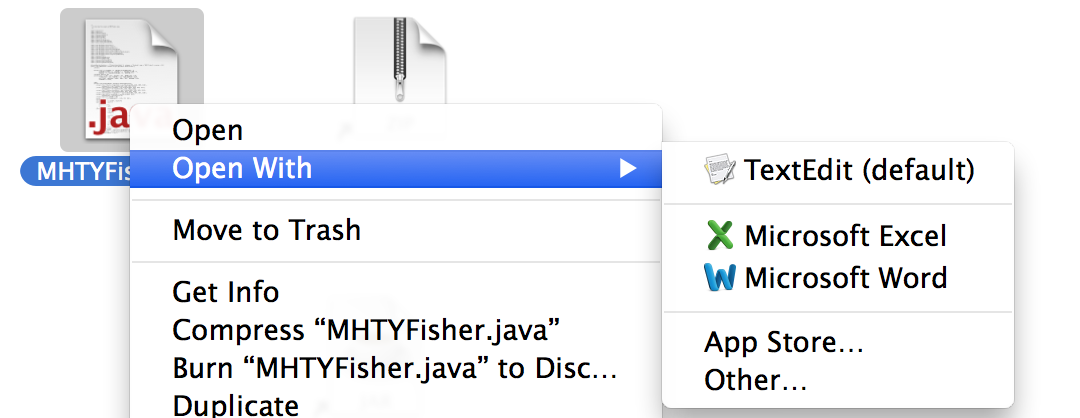This is a detailed screenshot of a computer screen with a white background, showing a right-click context menu. The image includes two icons in the background: one representing the file named "MHTYFisher.java" and another resembling a zipped document with a zipper down the middle. The name "MHTYFisher.java" is prominently highlighted in blue. The context menu displays various options, which include "Open," "Open With" (highlighted), "Move to Trash," "Get Info," "Compress 'MHTYFisher.java'," "Burn 'MHTYFisher.java' to Disk," and "Duplicate." An arrow points to another pop-up menu next to the "Open With" option, listing available applications for opening the file: "Text Edit (default)," "Microsoft Excel," "Microsoft Word," "App Store...," and "Other...".